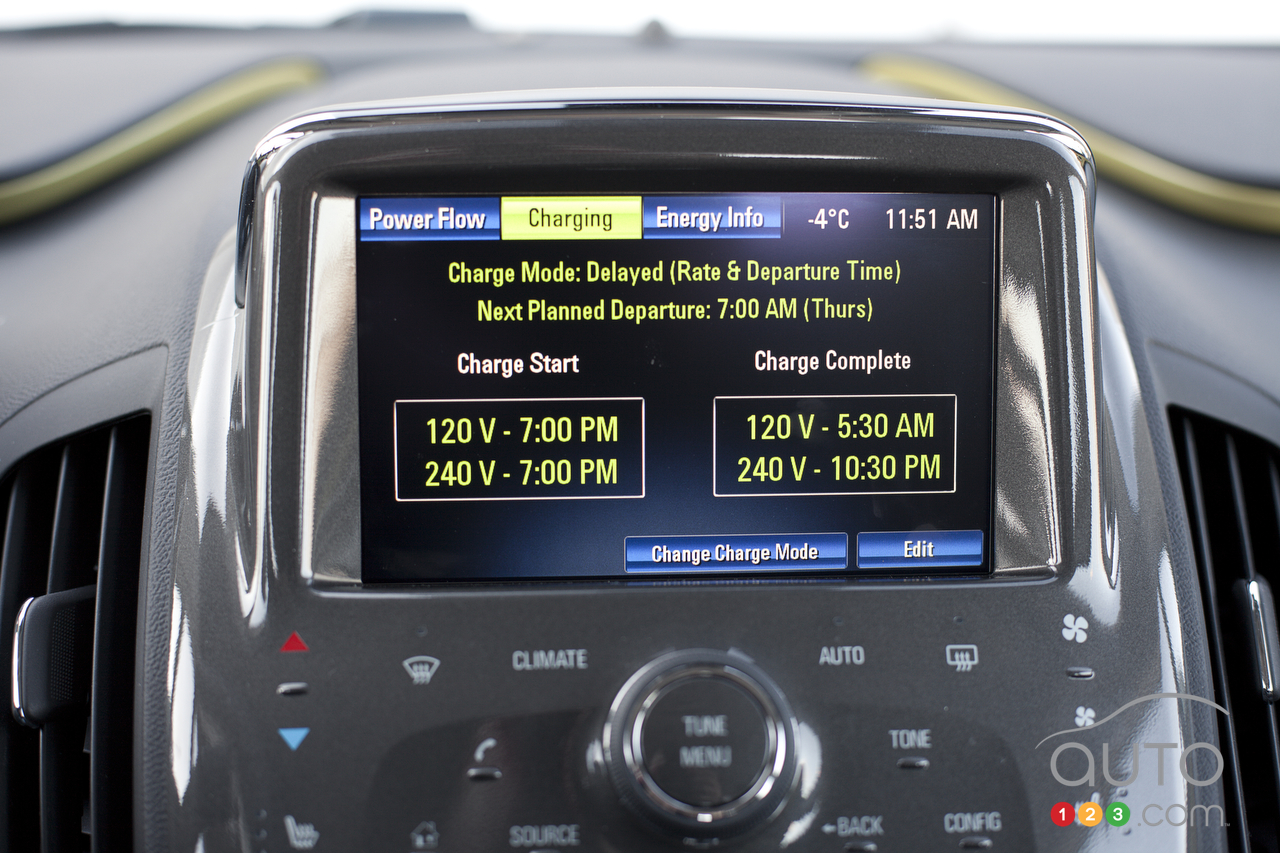This image showcases the central dashboard of a vehicle, featuring a prominent digital display flanked by heating and air conditioning vents on either side. The dashboard has a dark gray color scheme, with elevated sections on the top left and right, suggestive of airbag compartments.

Dominating the dashboard, the digital display's interface has a black background, adorned with tabs at the top labeled "Power Flow," "Charging" (highlighted in yellow), and "Energy Info." The top bar further displays the current temperature at -4°C and the time at 11:51 AM. Below these tabs, the screen details "Charge mode" set to delayed, along with "Rate" and "Departure time." The text indicates the "Next planned departure" is at 7:00 AM on Thursday.

In the middle section, the display outlines charging schedules: on the left, "Charge start" for both 120 volts at 7:00 PM and 240 volts at 7:00 PM; on the right, "Charge complete" shows 120 volts at 5:30 AM and 240 volts at 10:30 PM. Toward the bottom right, there are two buttons labeled "Change charge mode" and "Edit."

Beneath the digital display, the dashboard features standard climate control options including buttons for temperature adjustment (red for up and blue for down), defrost, auto, and fan speed. The central control area also includes a knob for tuning and accessing the menu, with a button in the middle labeled "Tune Menu." Additionally, a watermark at the bottom of the screen reads "auto123.com," hinting that this image may originate from an automotive information platform.